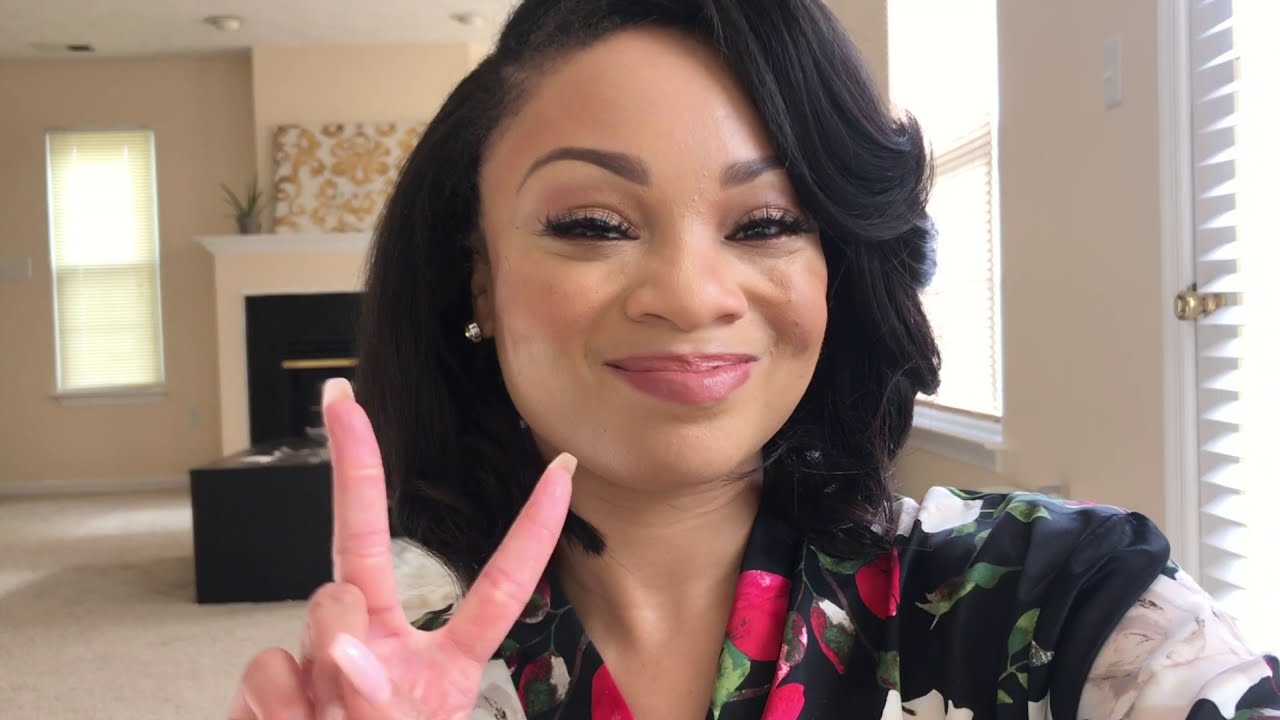The photograph is a horizontal, up-close selfie of a woman with short, wavy, black, shoulder-length hair, taken in a well-lit room that appears to be a living room. The woman has an elaborate makeup look, featuring fake eyelashes, curved brown eyebrows, eyeliner, and a dull pink matte lipstick accentuating her thick lips. She has studded earrings and pretty long fingernails. She is holding up her right hand in a peace sign, with her forefinger and middle finger extended. She wears a black floral-patterned dress with pink roses, green leaves, and white accents, cropped mostly at her shoulders. Her left hand holds the camera, adding to the selfie pose with her left shoulder slightly raised. The background reveals a cozy living space with a fireplace adorned with a picture frame and a plant on the mantle, a door with built-in blinds leading outside, light brown walls, a vertical rectangular window to the left, and beige-colored carpet flooring. The room is filled with natural light, giving it a bright ambiance.